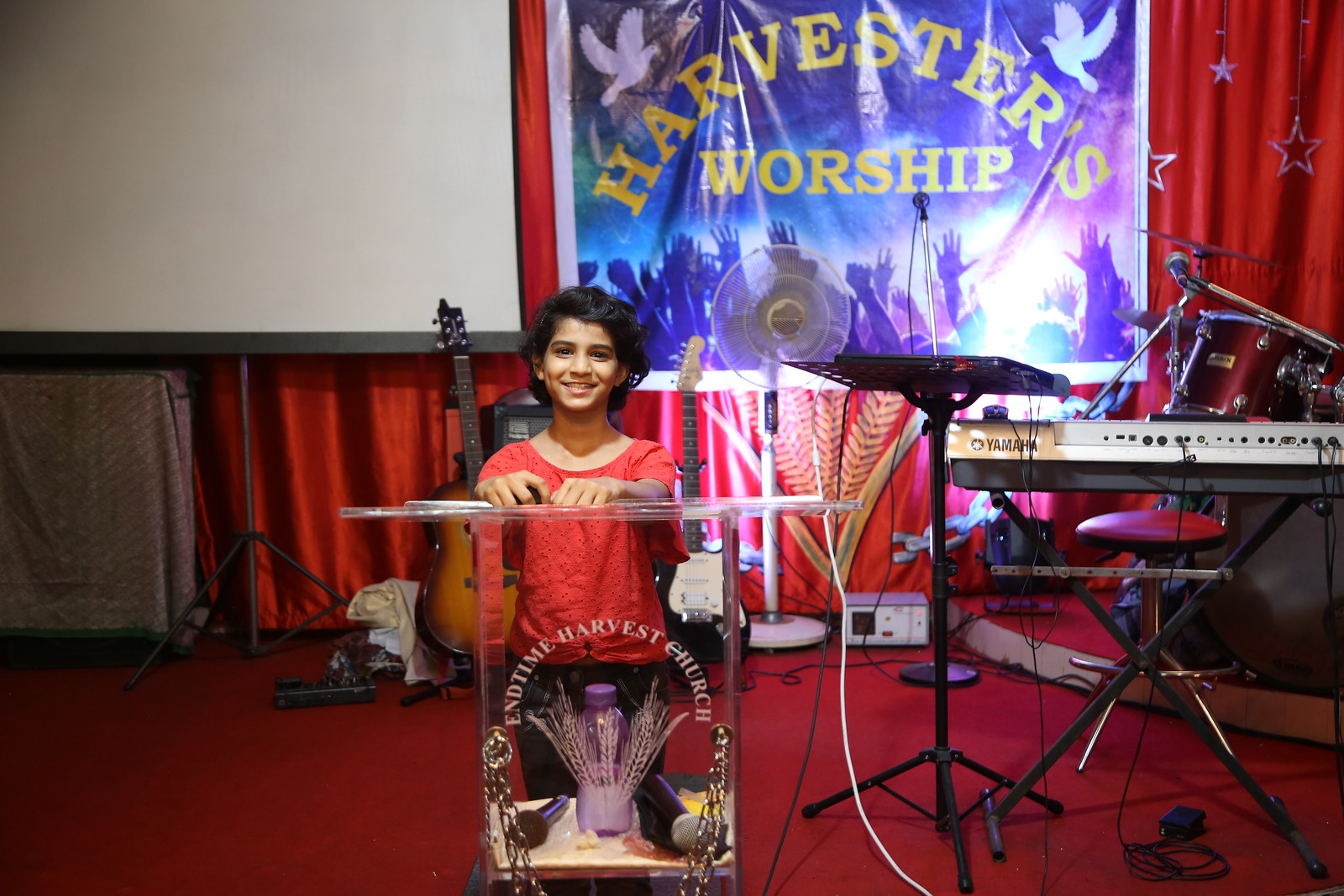Inside a church, a medium-length black-haired girl stands on a stage, smiling brightly. She wears a red t-shirt and is positioned behind a clear podium equipped with two microphones and a purple bottle of liquid. The podium bears the words "End Time Harvest Church." The stage, carpeted in red, is set against a backdrop of a red curtain adorned with stars and a banner that reads "Harvesters Worship," featuring doves and raised hands. Behind her, the stage is filled with musical instruments including a Yamaha keyboard, several guitars, and a drum set, alongside an amplifier and various wiring. A projector is mounted in the top left corner, casting over the musical setup, establishing the space as a dedicated area for church performances.